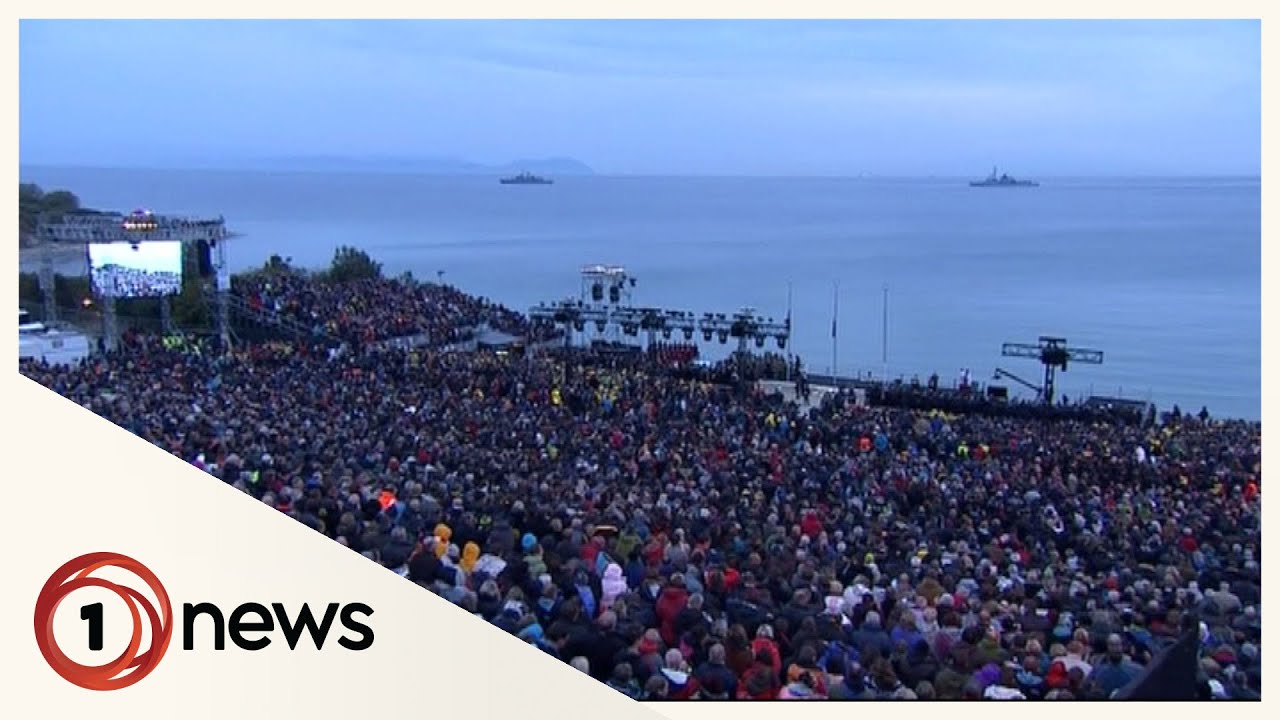This detailed photograph, possibly a screenshot from a local station labeled "Number One News" (with a red-circled '1' logo in the bottom left corner), captures a large crowd—potentially over 2,000 people—gathered along a waterfront. Attendees, many clad in jackets, hats, and rain gear suggesting colder weather, face towards the water where a concert or musical event appears to be taking place. Metal scaffolding that likely supports stage lights is visible at the water's edge, and a substantial jumbotron screen on the left side shows the scene to the crowd. The scene is set against a backdrop of a vast body of water at dusk, with two large ships anchored in the distance, creating a picturesque yet busy atmosphere.